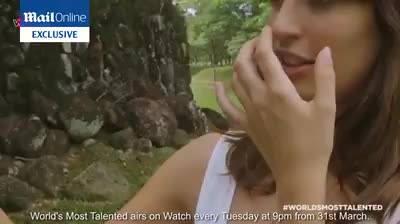This image appears to be a screenshot from a television program. In the upper right-hand corner, a blue and white text box reads "Mail Online Exclusive," although the precise wording may be slightly distorted or repeated. The scene features a young girl, only partially visible from just under her eyes to just below her shoulders, with her left shoulder cropped out of the frame. She has long brown hair and is wearing a white tank top. The girl seems to be talking or laughing, her left hand covering her mouth as if she's stifling a giggle. The background suggests she's in a park, featuring rock structures, trees, and green grass. At the bottom left corner, in white font, the text reads "#WorldsMostTalented" followed by "World's Most Talented airs on WATCH every Tuesday at 9 p.m. from 31st March." The overall image gives the impression of an engaging moment captured from a lively television show.